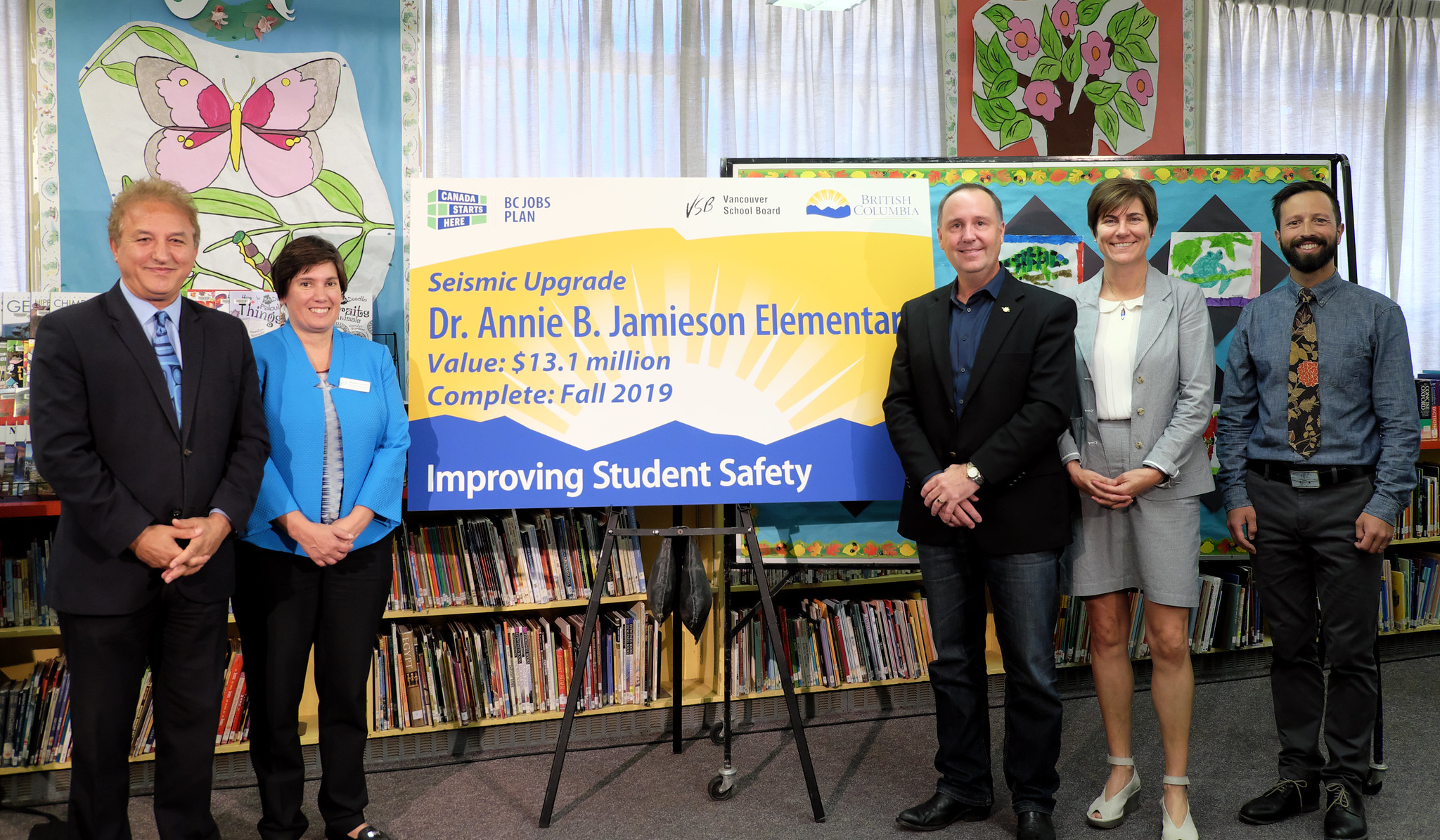In this color photograph taken in a library, five people pose surrounding a large rectangular sign on a black tripod. The room features white curtains, a gray floor, and shelves full of books. The background displays several pastel-colored drawings, including one depicting a butterfly and another with a tree adorned with pink flowers. The sign is prominently white at the top, yellow in the middle, and blue at the bottom, with text that reads, “Seismic Upgrade Dr. Annie B. Jamieson Elementary, value $13.1 million, completed Fall 2019, Improving Student Safety.” On the left side of the sign stands a man in a black suit and blue tie, next to a woman in a turquoise jacket with short hair and black pants. On the right, there is a man in a black suit jacket and blue shirt, a woman with short hair wearing a gray jacket and gray shorts, and a man with a beard and mustache dressed in a green shirt, black pants, and a colorful floral tie.